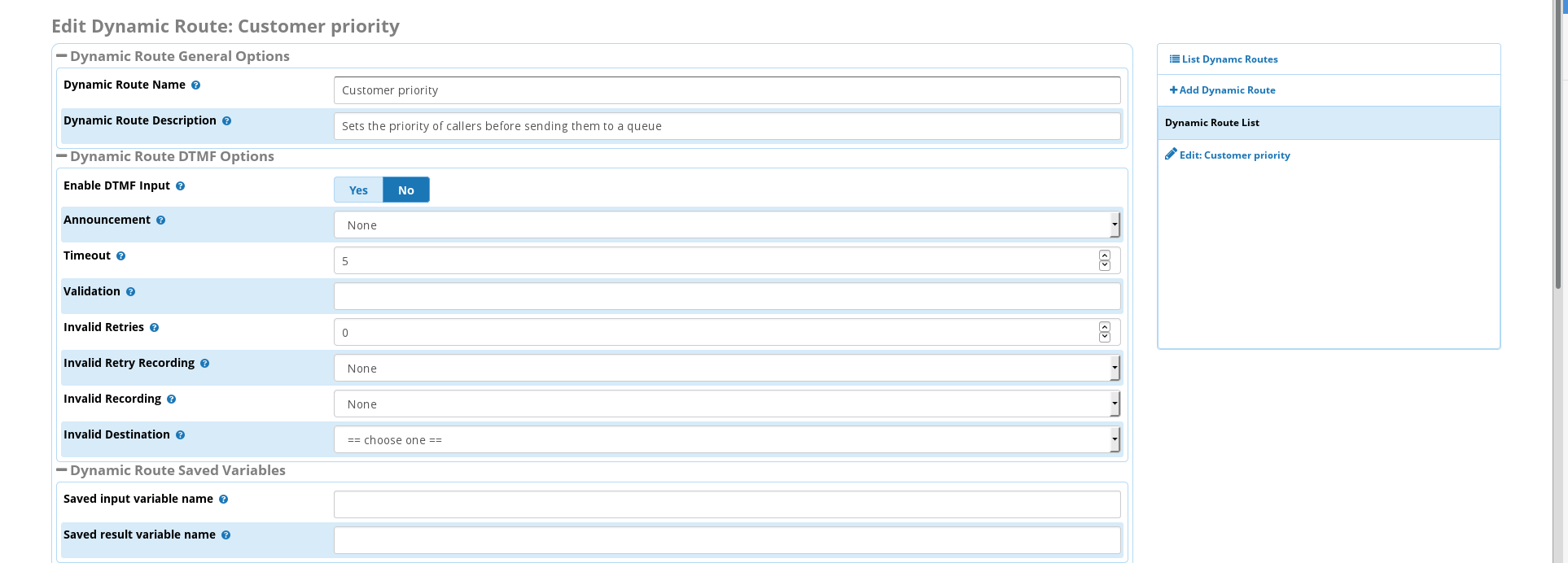**Descriptive Caption:**

Screenshot of the "Edit Dynamic Root Customer Priority" options page, likely used for managing deliveries or server operations for a business like FedEx or the United States Postal Service. The interface features a visual layout with alternating bars of light blue and white background and black text.

At the top of the page, under "Dynamic Root General Options," fields for "Dynamic Root Name," "Custom Priority," and "Dynamic Root Descriptions" are provided. A note explains that this page can set the priority of callers before sending them to a queue.

Beneath this section is "Dynamic Root DTMF Options," where the "Enable DTMF Input" option is set to "No" in dark blue with white lettering, though there is a "Yes" option available in dark blue with a light blue background. Additional settings include "Announcement: None," "Timeout: 5," "Validation: Not put in," "Invalid retries: 0," "Invalid retry recording: None," "Invalid recording: None," and "Invalid destination" with an option to choose one.

The page also presents "Dynamic Root Saved Variables" with fields for "Saved Input Variable Name" and "Saved Result Variable Name."

On the right side of the interface, a menu provides options such as "List Dynamic Roots," "Add a Dynamic Root," "Dynamic Root List" (displayed in black), and "Edit Customer Priority," with other options in light blue, indicating clickable hyperlinks.

Overall, the screenshot depicts a root management system that appears suitable for delivery services or similar logistical operations.